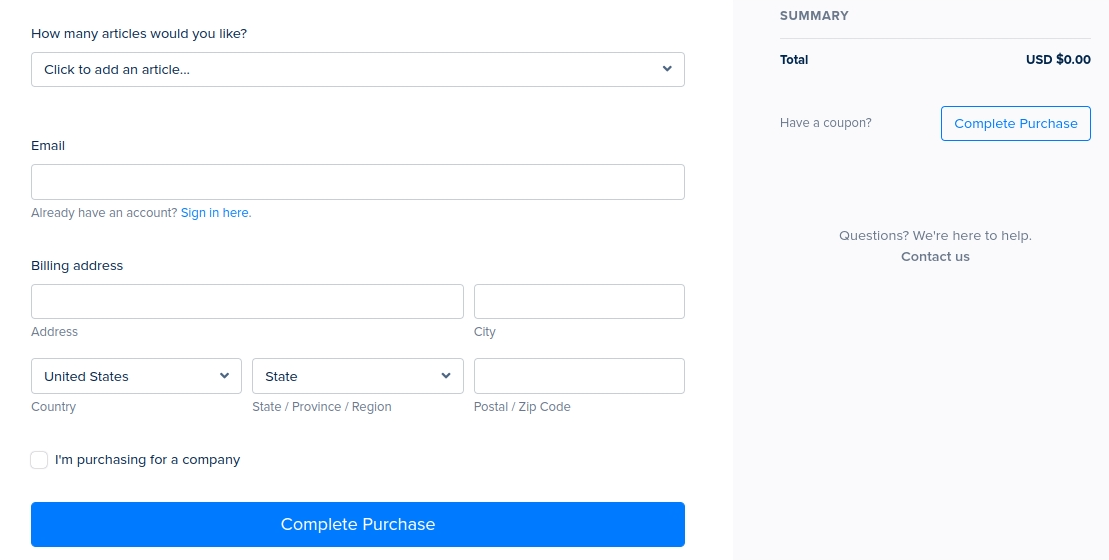**Detailed Caption:**

The screenshot depicts a checkout page on an unidentified website. The checkout interface is split into two main panels. The left panel, which occupies roughly two-thirds of the screen, consists of various form fields for user input. Here, users can specify the number of articles they wish to purchase in a rounded rectangle dropdown menu labeled "How many articles would you like?" Below, there is a blank email field also encased in a rounded rectangle. To the right of this field is a prompt indicating, "Already have an account? Sign in here," with "Sign in here" highlighted in blue to denote a hyperlink.

Further down in the left panel, there are fields for billing information: empty fields for address and city, with "United States" pre-filled in the country dropdown menu, and a completed state/province/region field. The postal or ZIP code field is left blank. Additionally, there is an unchecked checkbox option labeled "I'm purchasing for a company."

The right panel, occupying one-third of the screen, has a subtle gray background and displays the order summary. At the top, a bold header reads "Order Summary" followed by a line showing a current total of "USD 0.00". Below, there is an option to apply a coupon, and a prominent blue-outlined, rounded rectangle button labeled "Complete Purchase" in blue text. Below this button, in smaller gray text, it reads "Questions? We're here to help," with "Contact us" in a slightly darker gray font indicating it may be a hyperlink.

At the very bottom of the page, there is another blue rounded rectangle button with "Complete Purchase" written in a white font.